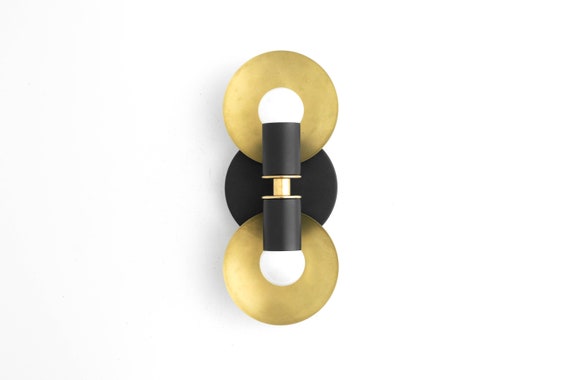This image features an elegant, modern wall sconce mounted on a plain white background, highlighting its three-dimensional form through its shadow. The sconce comprises three flat circular plates arranged vertically, much like a snowman, with a black circle sandwiched between two gold circles. Each gold circle resembles a washer, adding a sophisticated touch to the fixture. Protruding from the center of these circular plates is a series of cylindrical elements: two black cylinders with gold trim at the top and bottom, connected by a smaller gold cylinder in the middle. Each end of the larger black cylinders features a luminous spherical bulb that aligns perfectly within the gold circular plates, creating a striking contrast. The top and bottom illuminated spheres add to the fixture's fancy and elegant appearance, emphasizing the black and gold color scheme that mingles traditional and modern design elements beautifully.